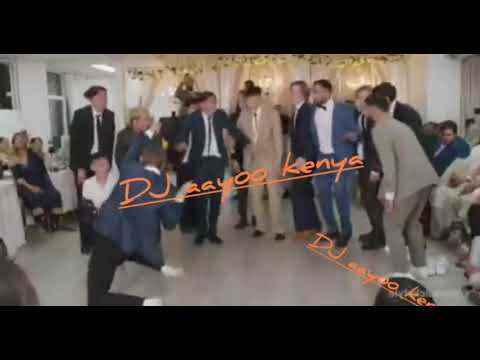This image captures a joyous event, likely a wedding or ceremonial dance, featuring a group of men dressed in various colors of suits including black, tan, and shades of blue. They are on a white-tiled open floor space, energetically dancing or performing, with one standout figure in a blue suit facing the group. Surrounding them, on the right and left edges, are seated guests at tables draped in white tablecloths, observing the lively scene. The backdrop includes white walls adorned with possibly lace curtains, softly illuminated from above. Cutting across the center of the image and repeated in the bottom right corner in diagonal orange text is the phrase "DJAA YOO Kenya." The picture is framed by black bars at the top and bottom, suggesting a widescreen format. Despite its low resolution, which renders the faces indistinct, the image vividly conveys the spirited ambiance of the celebration.